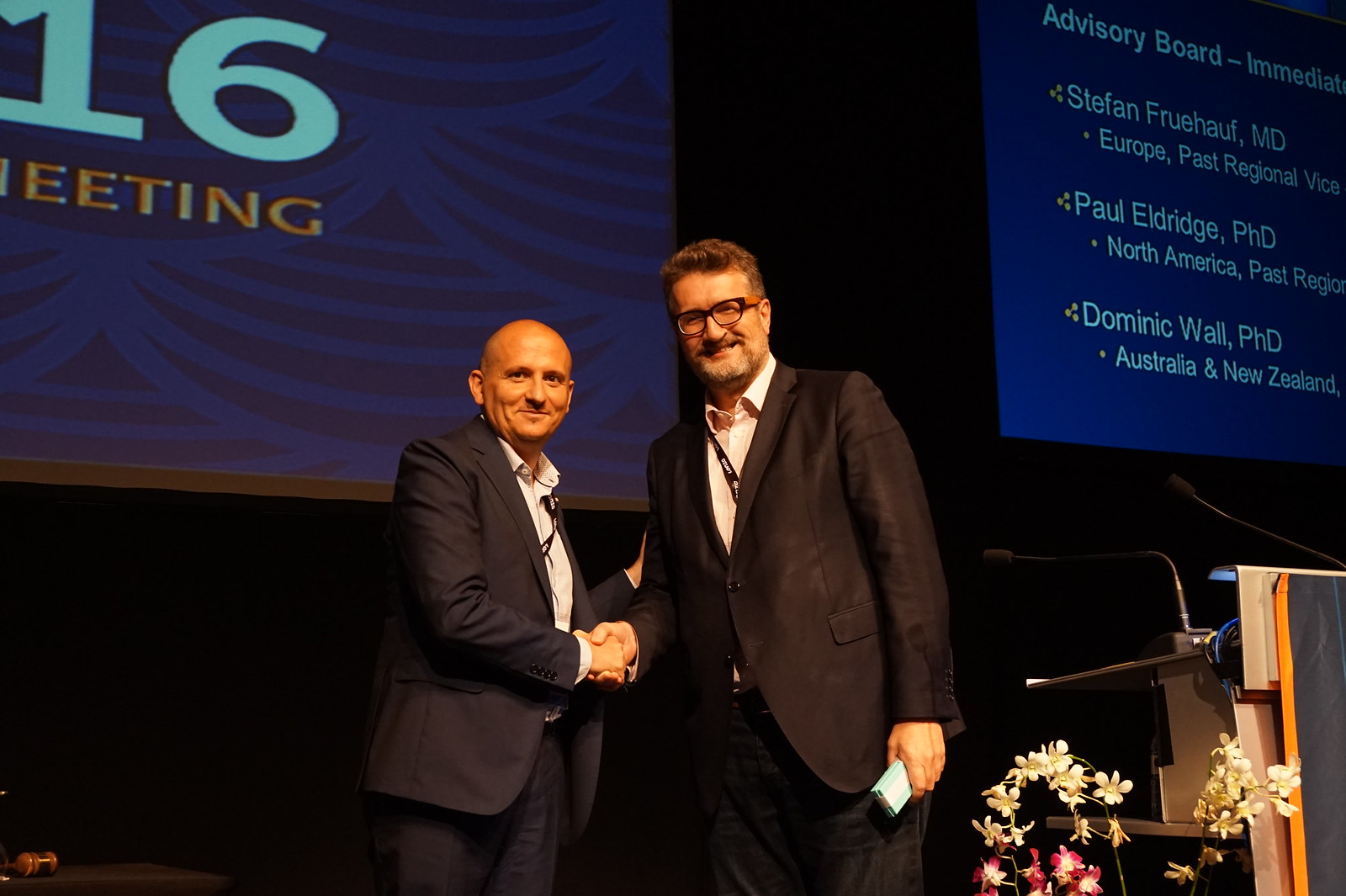In the photograph, we see two men standing side-by-side on a stage, shaking hands and smiling at the camera. Both are dressed in black business suits with white collared shirts underneath. The shorter gentleman on the left is bald, while the taller individual to the right has a few inches of black hair and is wearing black glasses. The taller man is also holding a blue box in his left hand during the handshake. Behind them, two projector screens display fragmented text; the left screen partially reads "16 meeting," and the right screen mentions "advisory board" with names such as Stefan Fruhall, MD; Paul Eldridge, PhD; and Dominic Wall, PhD. Their respective regions of Europe, North America, and Australia/New Zealand are also noted. Adjacent to the men is a podium with microphones, and white flowers adorn the left side of the stage. The scene suggests a formal event, possibly an award presentation, given the professional attire and setup.